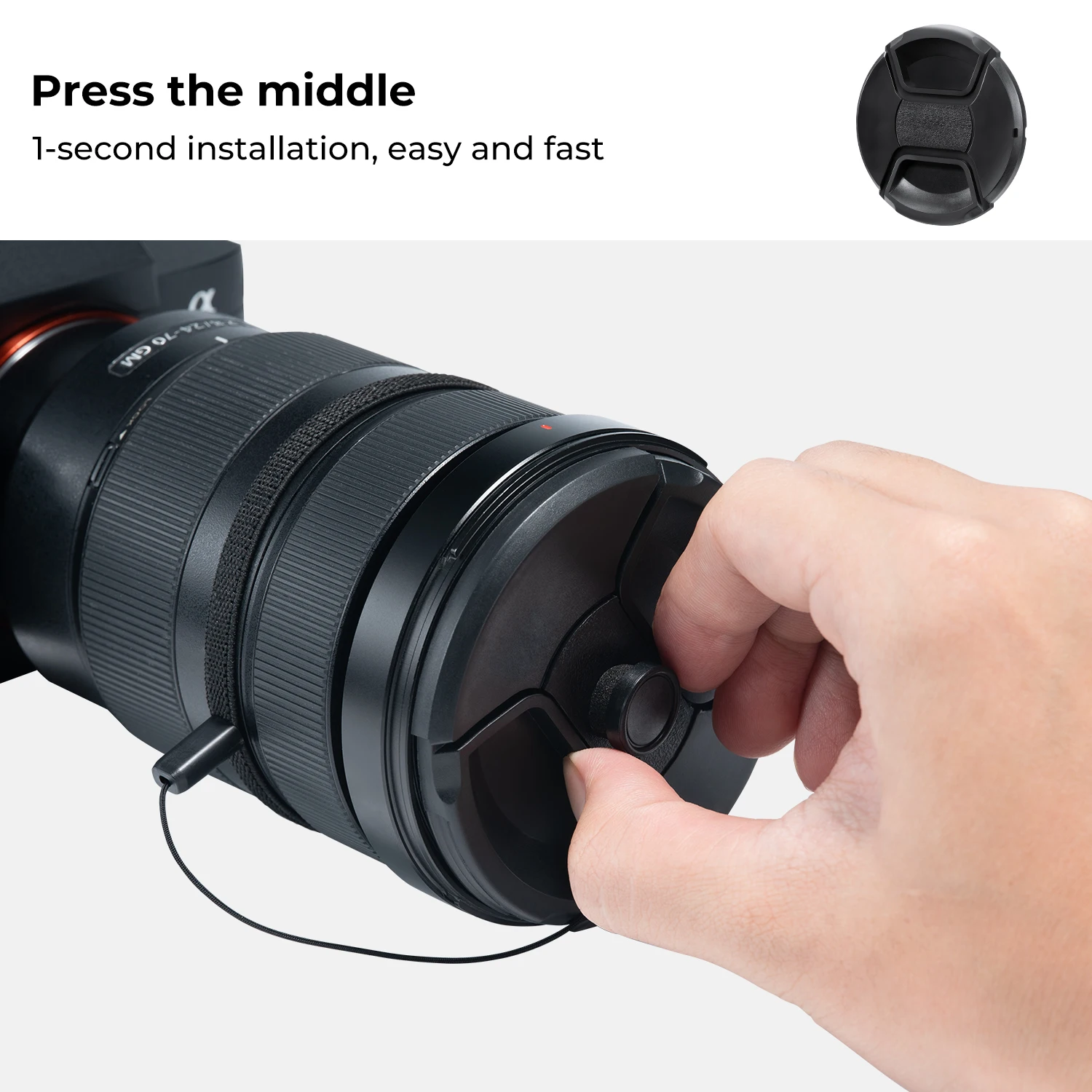The image presents a clear, instructional advertisement for a camera lens cap accessory against a very light gray background. At the top, there is a rectangular white box containing black text that reads "Press the middle. One second installation, easy and fast." Below this text, the focus is on a large black camera, presumably a Sony Alpha, fitted with a long telephoto or zoom lens. The lens cap is black, thin, and circular, shown being attached to the lens by a hand. This cap is connected to the camera via a small black string, which is secured to the lens with a Velcro or elastic strap, featuring a plastic post. The overall scene illustrates the simplicity and convenience of installing the lens cap, emphasizing its quick "one second installation."